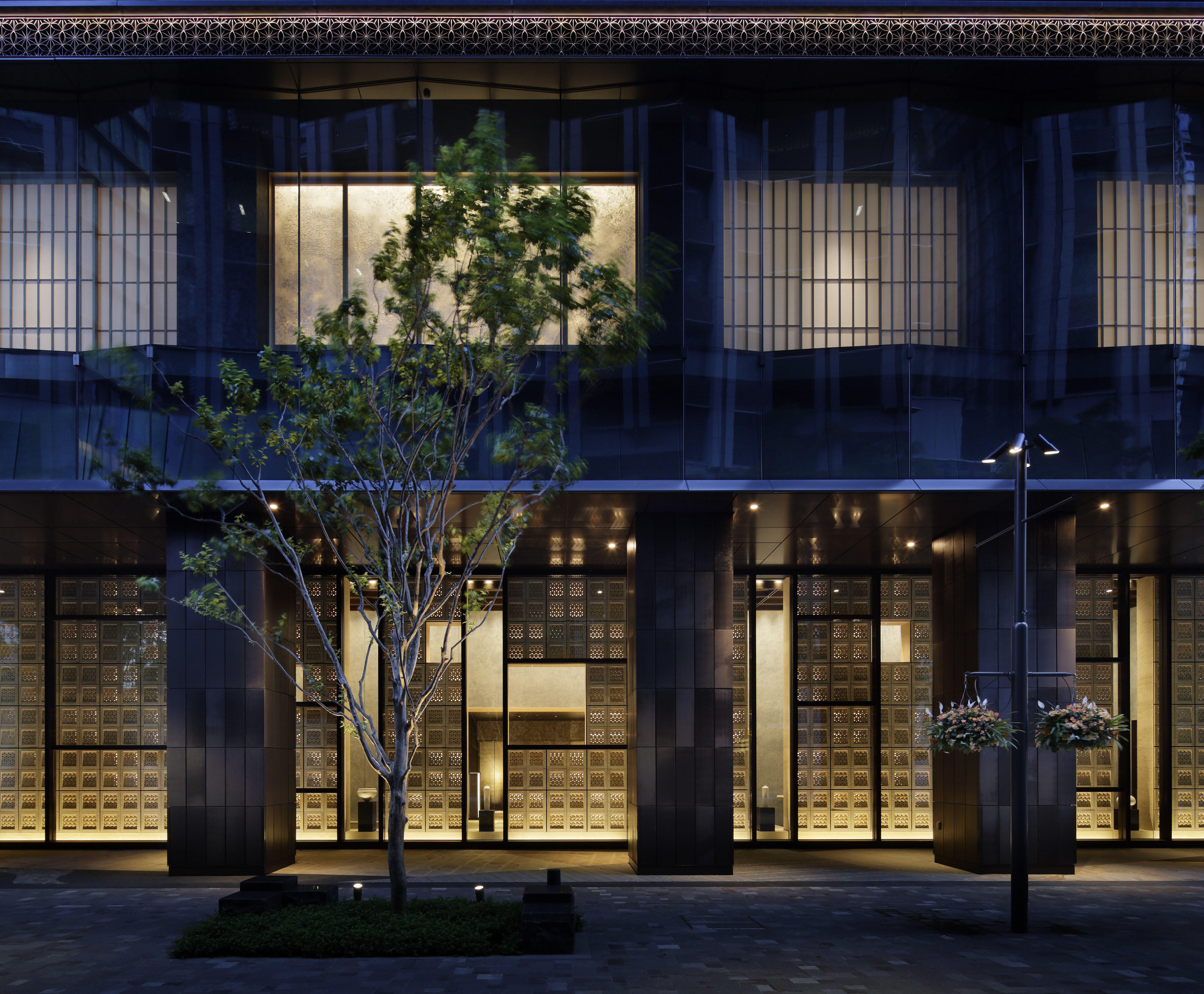The image showcases a contemporary and modern building with a distinctly Asian-inspired architectural style, situated within an urban environment. The exterior walls of the building are adorned with glass windows featuring intricate cubic patterns that give the facade an opaque and stylish look. The structure boasts a blend of golds, grays, and whites, delivering a clean and sophisticated aesthetic. 

Amidst cobblestone or brick pavement, a prominent tree stands in the foreground, its base highlighted by two spotlights, emphasizing its presence against the night sky. Adjacent to the tree, a lamppost with hanging flower baskets, bursting with muted greens and purples, adds a touch of nature to the otherwise urban scene. The photograph, taken at night or dusk, captures the warm, golden glow emanating from the illuminated interiors of the building's first floor, contributing to the calm and serene ambiance of the setting.